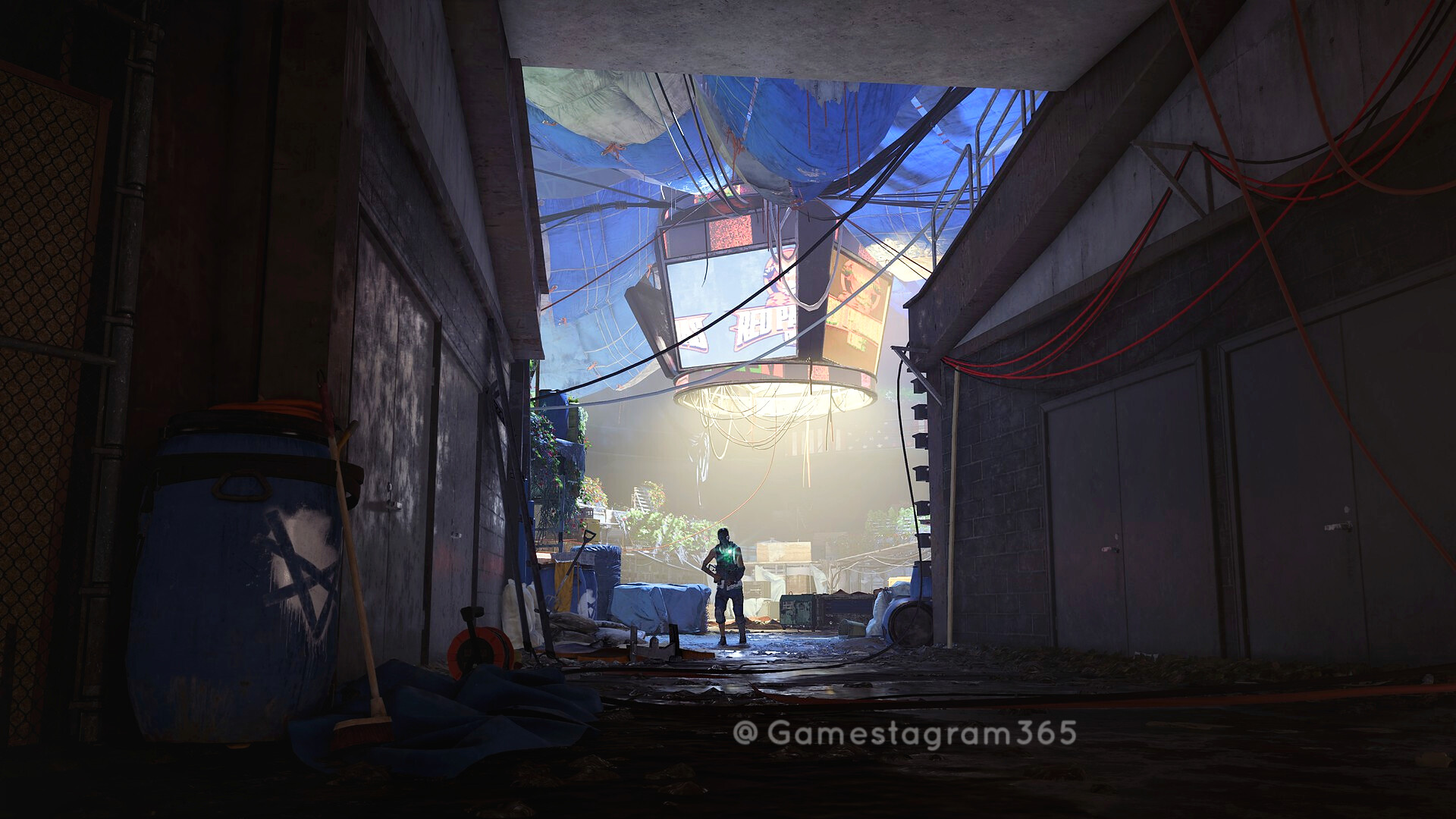This screenshot from a video game, possibly concept art or a drawing, showcases a vivid and colorful image of an arena similar to Madison Square Garden. At the center stands a man beneath a large, square scoreboard that tapers at the bottom and emanates wires and light from a circular base. Surrounding the arena are various dark gray walls, with lighter shades of gray and brown showing wear and tear. To the left, there is a brown trash can with a black bag, an orange and black cylinder on the floor, puddles of water reflecting the light, a shovel, and a light brown cylindrical pole. To the right, the scene features red cords strewn about, two sets of closed double doors with silver handles, and additional gray shading near the roof. The upper section of the arena includes a titan-tron like display and various hanging wires. Green plants and remnants of the stadium add to the detailed and immersive environment. The bottom of the image contains a watermark reading "GameStagram365."